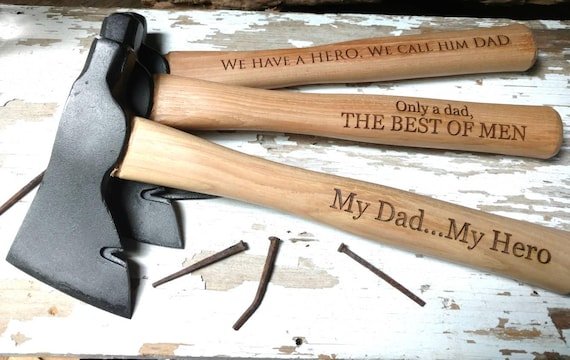This image depicts a weathered workbench with peeling white paint that reveals the underlying brown wood, underscoring its age and usage. The centerpiece of the scene features three small axes, each with a dark metallic head and a wooden handle. Scattered around the axes are four rusty, flat nails, one of which is bent, suggesting they are old and no longer usable.

Engraved on the handles of the axes are heartfelt messages:
1. The first axe, positioned at the bottom of the stack, bears the inscription, "We have a hero. We call him Dad," etched in all capital letters.
2. The second axe, resting atop the first, states, "Only a Dad, The Best of Men," with the latter part also in all capitals.
3. The third axe, placed on top of the other two, reads simply, "My Dad... My Hero," in standard lettering.

These inscriptions highlight a theme of paternal respect and admiration, making the tools both practical implements and sentimental keepsakes.